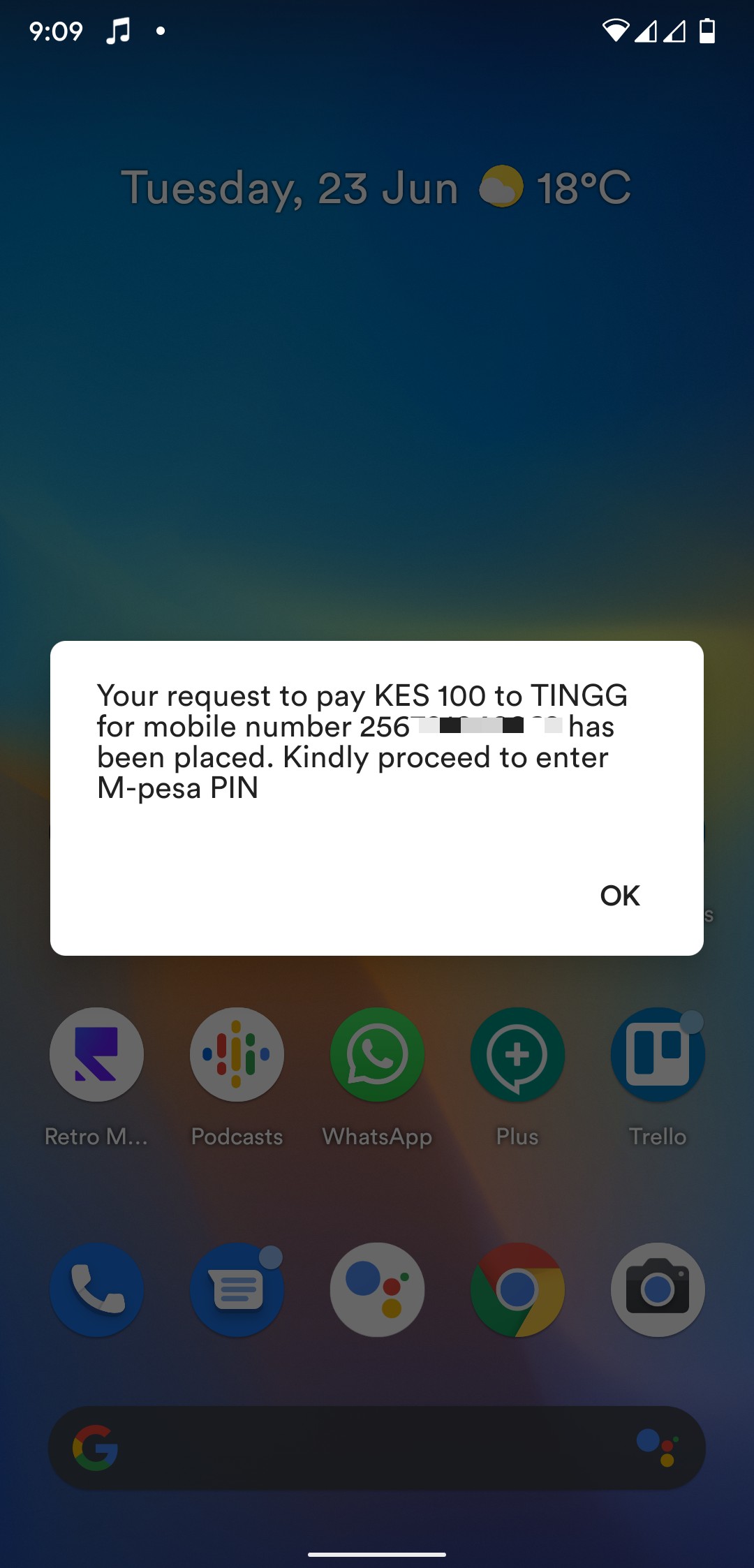The image depicts a smartphone screen at 9:09, though it's unclear whether it's morning or night. The battery level is approximately half full. The background shows the date as Tuesday, 23 June, with a partly cloudy weather icon indicating a temperature of 18 degrees Celsius. A pop-up notification prompts the user to enter their M-PESA PIN to complete a payment of KES 100 to TINGG for a mobile number, which is partially obscured for privacy. The notification includes an "OK" button to confirm the transaction. Behind the bright pop-up, the dimmed wallpaper reveals various app icons, including Metro M, WhatsApp, Trello, Phone, Text, Google Chrome, and Camera.